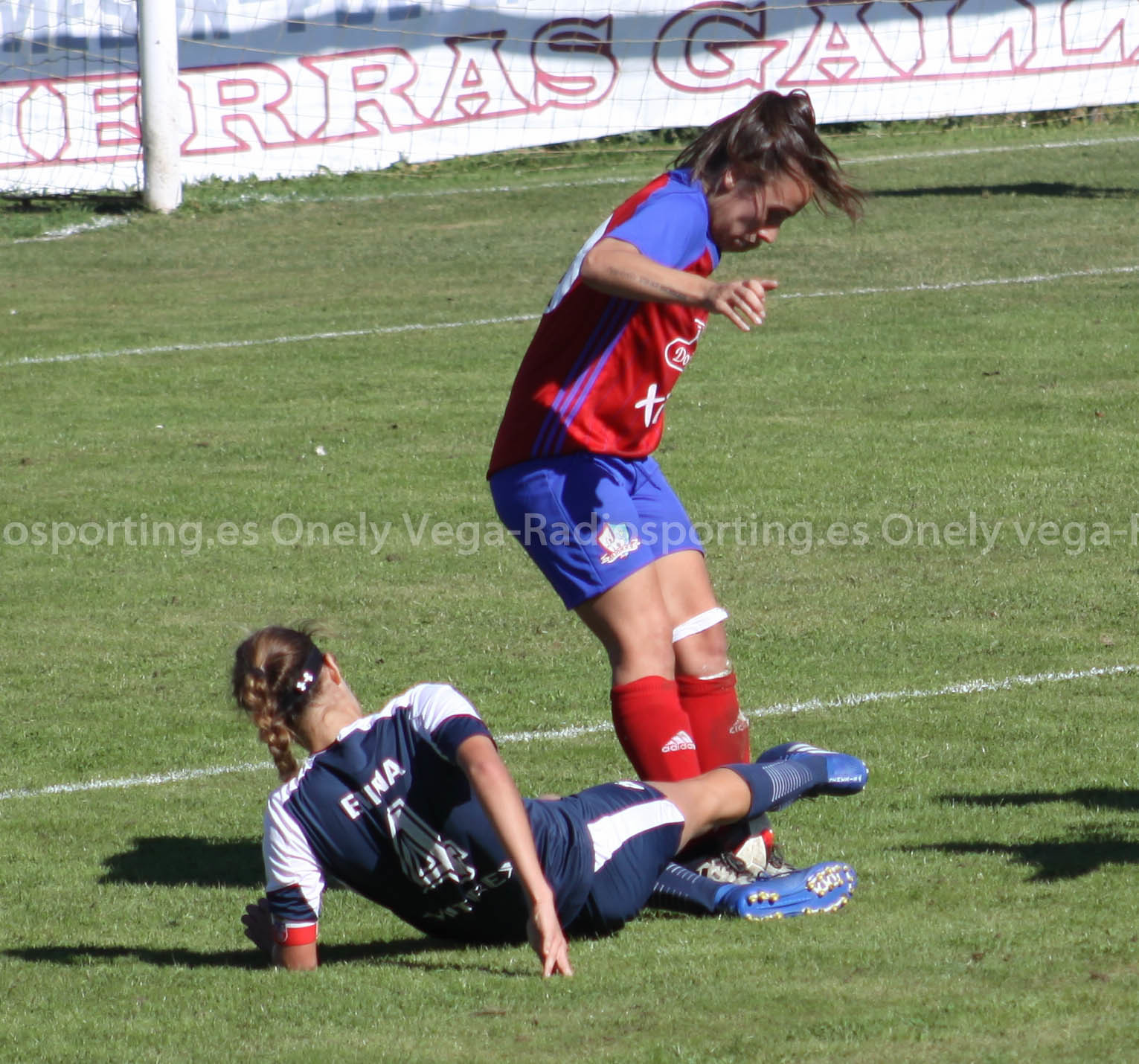This is a detailed photograph capturing a dynamic moment between two women on a soccer pitch. The woman standing is wearing red socks, blue shorts, and a red and blue top, appearing to be part of the Doncaster Rovers team. She is attempting to kick the ball, which is wedged between her ankles. Her opponent, identifiable by the number 4 on her dark blue and white striped shorts and matching top, is lying almost horizontally on the ground with her hair braided and pulled back. Her leg is entangled with the ball, adding to the intensity of the contest. The scene is set against a backdrop featuring a white sign with partially red and white writing, likely indicating sponsorship or team details. The soccer pitch itself is marked by white lines and scattered shadows. Superimposed text across the center reads "sporting.es, Onale, Vega, Radisporting.es," suggesting a publication or watermark.